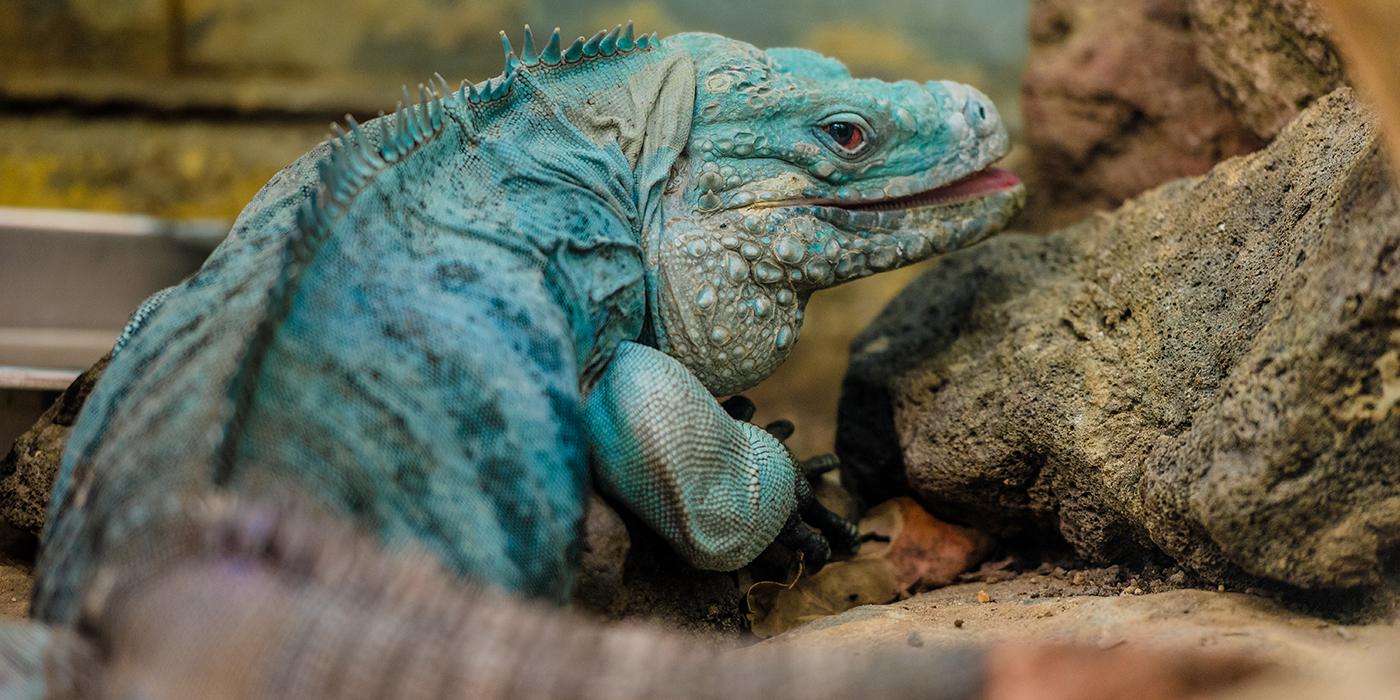In this detailed photograph, a striking blue-green iguana, possibly a blue iguana, is prominently featured in a natural, grassland environment, bathed in daylight. The iguana, positioned with its back end facing the camera and heading towards the back of the image, has its head turned towards the right. It exhibits a beautiful aqua color on top with a light yellow-beige underside, transitioning to a brown tail curving to the right corner of the image. This tail and part of its body create a blurred effect due to movement. The iguana's chin rests just above a light brown, grayish rock, and its eye, a mix of black with a tinge of brown on the right side, glimmers with a red hue.

Notably, the iguana's neck and head are adorned with circular bumps, and spikes, matching its seafoam green-blue hue, run along its back. Its surroundings are dotted with earthy-colored rocks—tan, brown, and hints of green—accentuating the reptile's vibrant coloration. The iguana's open mouth and the intricate details of its scales add a dynamic and lifelike quality to the scene.